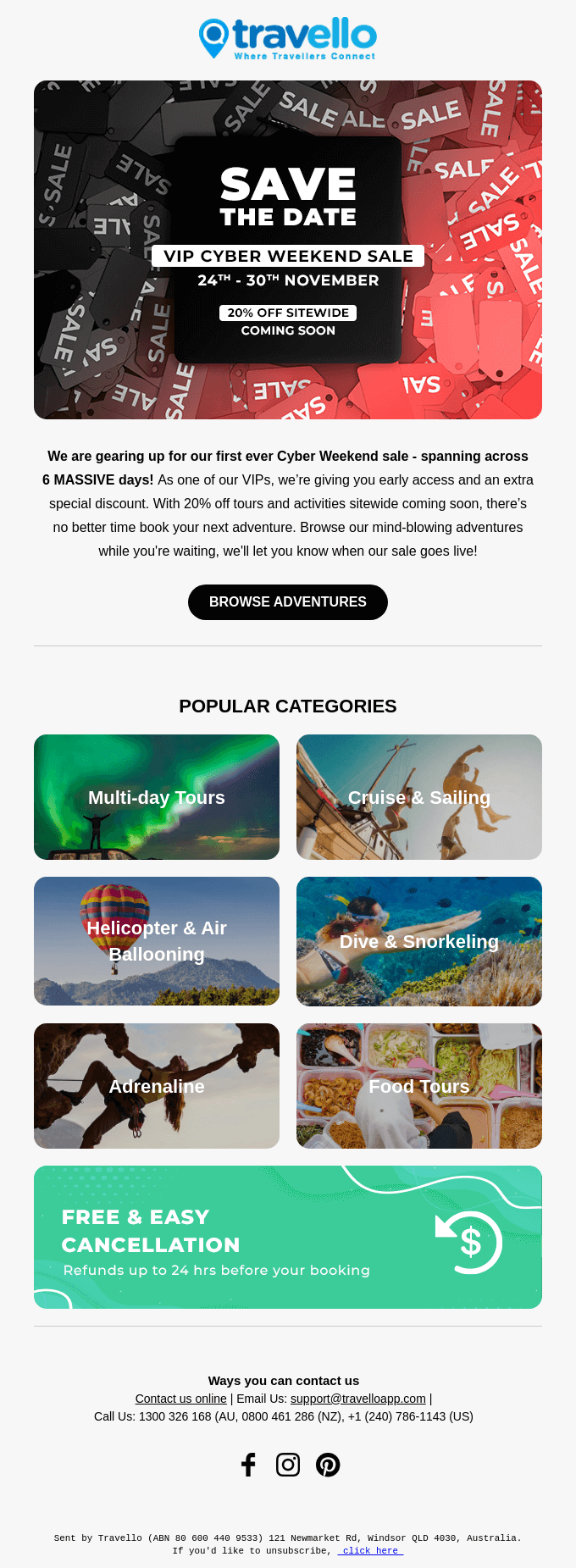A promotional image for Trevello, targeting potential travelers with an announcement for an upcoming VIP Cyber Weekend Sale. This vibrant graphic, likely sourced from a smartphone screenshot, highlights a compelling offer of "20% off sitewide," urging customers to "Save the Date." Trevello, a booking platform for various travel experiences such as vacations, mini-travel destinations, multi-day tours, helicopter and air tours, ballooning, adrenaline-packed activities, food tours, diving, snorkeling, and cruises, also emphasizes its flexible cancellation policy with a green section at the bottom of the image depicting a dollar sign and a counter-clockwise arrow.

The image features a clean white background with vibrant, multi-colored thumbnails representing popular categories, each neatly displayed in grids of either four or six images. Key information, including details about the Cyber Weekend Sale, is prominently highlighted in a color palette of black, red, and white. The browsing section remains slightly obscured, but the Trevello brand stands out in blue, ensuring it's easily recognizable for potential customers.

Overall, this engaging announcement leverages colorful icons and clear, concise messaging to attract attention and drive bookings during the promotional period.